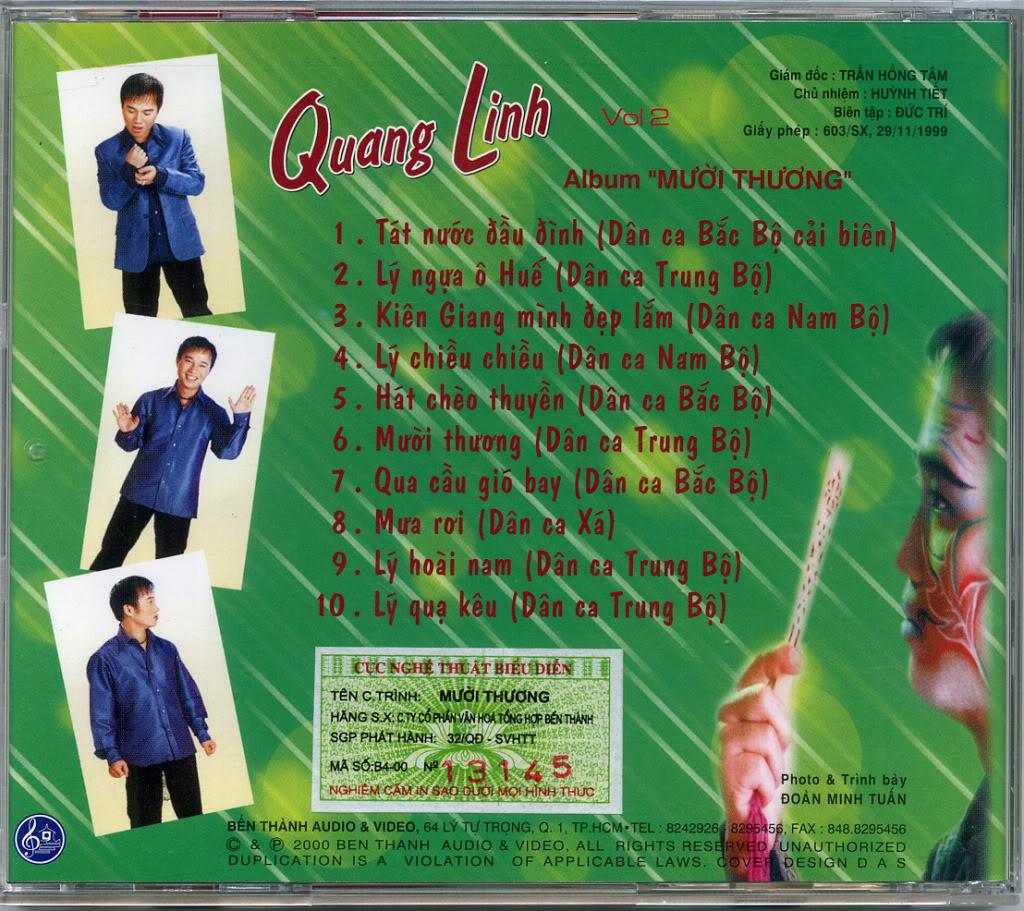The image appears to be the back cover of a plastic CD case with a vibrant green background and red text. It prominently features the name "Quang Linh, Volume 2, Album Muoi Thuong" at the top. Below the title is a list of ten song titles, all written in a different language.

On the left side of the cover, there are three somewhat crookedly placed photographs of an Asian man, presumed to be Quang Linh. The top photograph shows him looking down at his hands, seemingly adjusting his shirt cuff. In the middle photo, he is smiling directly at the camera while making a waving gesture. The bottom photo has him looking off to his left, as if gazing into the distance.

Additionally, there is an artistic, partial side-profile image of Quang Linh in the lower right part of the cover. This image has surreal elements, such as a red leaf pattern painted on his face and what appears to be the side of a handheld fan held in front of his face. This artistic photo also includes what looks like a magic wand. Throughout the cover, there is some contact information listed in the upper right corner.